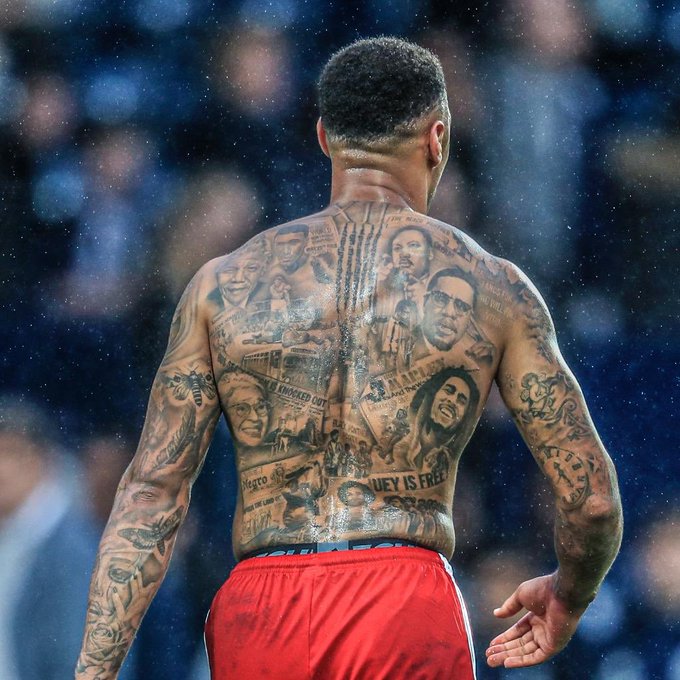The photograph captures an African-American man, shirtless and wearing red shorts with an elastic waistband partially revealing black underwear with text, possibly part of athletic attire. His short, curly hair is visible, alongside his upper body, which is extensively adorned with detailed tattoos. These tattoos prominently feature influential figures in black history: Martin Luther King Jr. on his upper right shoulder, Malcolm X below him on the lower right shoulder, Bob Marley in the lat region, and Rosa Parks on the left side. Nelson Mandela's image is situated across from Martin Luther King Jr., and there's a knockout image of Muhammad Ali, possibly hinting at Ali’s famous “float like a butterfly, sting like a bee” phrase, explained by additional tattoos of plants, bees, butterflies, and roses on the man's arms. Further embellishing his arms are various scrolls, clocks, and a cherub. The backdrop shows a blurry, indistinct crowd, suggesting an outdoor setting, possibly a sports event. The man stands centrally in the frame, walking away from the camera, making the entire focus on his tattoo-covered back and arms.